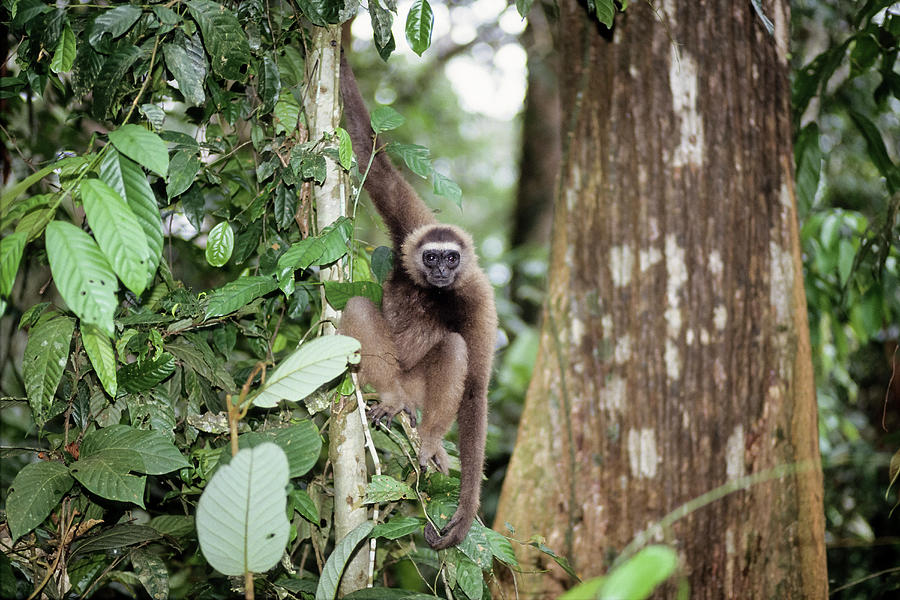The photograph captures a vibrant tropical rainforest setting with a diverse array of green leaves, vines, and trees. At the center of the image is a small-statured, furry monkey, most likely a Gibbon, showcasing its striking physical characteristics. The monkey exhibits a rich brown mahogany color with a unique white fur "crown" encircling its head and contrasting darker facial fur. The monkey's long arms and legs are well-displayed as it hangs from a slender tree trunk, gripping it with one hand while its feet rest against the foliage. The tree to the left is lush with green leaves and vines, while the tree to the right is a larger, more robust trunk marked with patches of missing bark and pale green or gray areas. In the background, additional trees and leaves are visible, along with glimpses of the sky peeking through the dense canopy. The overall color palette of the image is dominated by earthy greens, browns, and whites, emphasizing the natural beauty of the rainforest and its inhabitants.